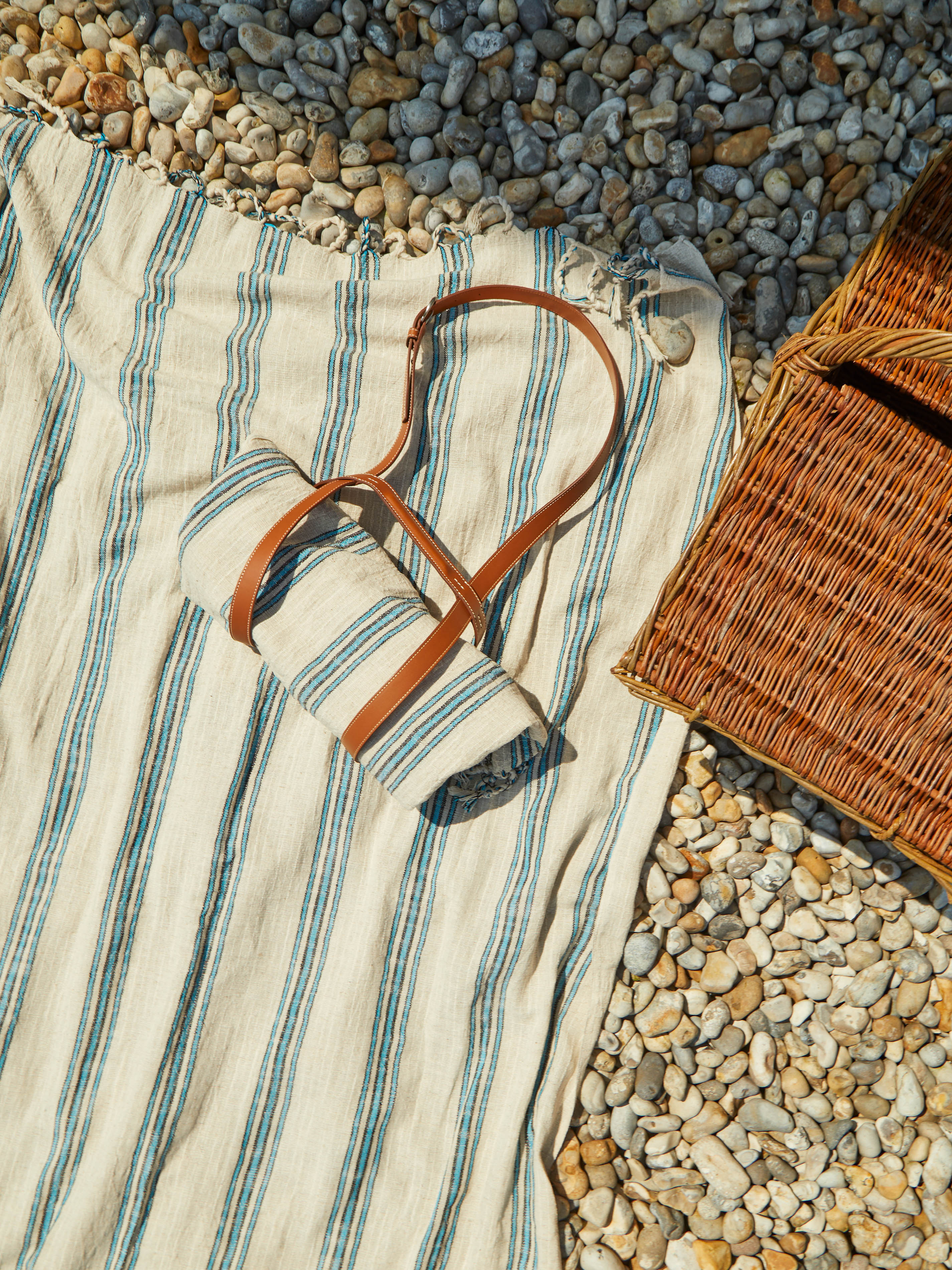A tranquil pebble beach stretches out in the photograph, with an array of smooth stones in shades of light grey, beige, yellow, and black forming a natural mosaic. Dominating the left side of the image is a large beach mat, positioned diagonally from the bottom left to the center. The mat is a murky white color, and a brown strap holder is neatly secured at its top right corner, suggesting it can be conveniently rolled up and carried. Placed adjacent to the mat on the right is a wicker picnic basket. The bottom left edge of the basket is visible, leading up to a sturdy handle that arcs upwards and vanishes off the right side of the image. Above this serene setup, a shadow sweeps across from just past the top left corner, casting a gentle, cool contrast over the warm hues of the pebbles below.